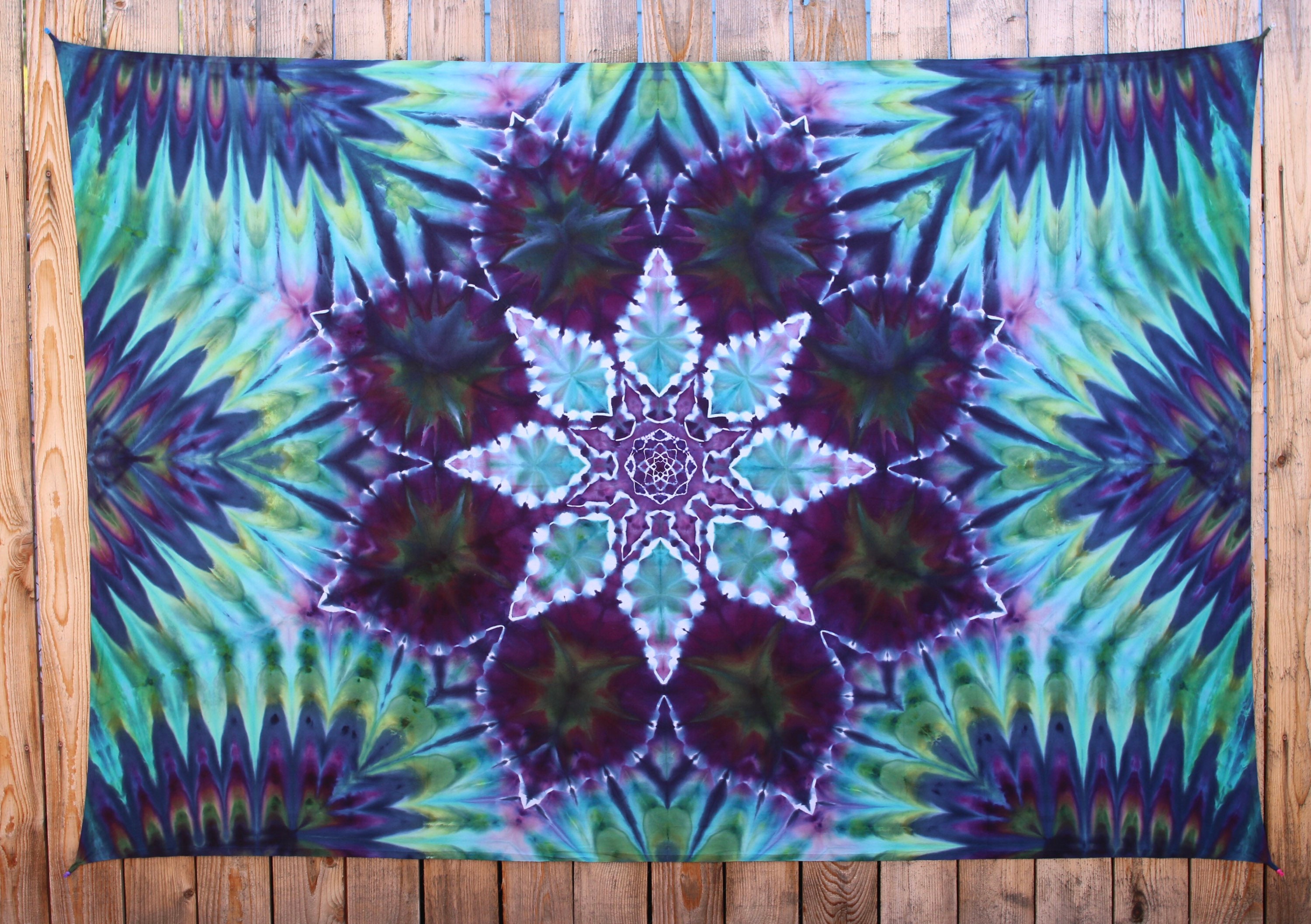The image is a horizontally aligned rectangular picture depicting a colorful sheet, flag, or blanket pinned against a fence composed of medium brown vertical wooden planks. The planks have gaps between them through which a blue sky is visible at the top. The sheet has a captivating tie-dye design featuring intricate patterns and vibrant colors. 

At its core is a large, central motif resembling a flower or snowflake with eight petal-like spikes. The petals radiate from a star-shaped center, which is predominantly light purple, bordered by darker shades of purple, almost appearing black. Surrounding this central figure are additional leaf or petal shapes in hues of green, teal, dark blue, and dark purple.

The edges of the sheet are adorned with more leaf designs, presenting a consistent pattern with blue and green-tipped leaves interspersed with lighter purple. The entire design displays a remarkable symmetry and vivid coloration, with the dominant colors being purple, blue, and green, and subtle touches of yellow. The sheet is secured to the fence possibly with thumbtacks, as indicated by red and blue spots in the lower right and upper left corners, respectively.